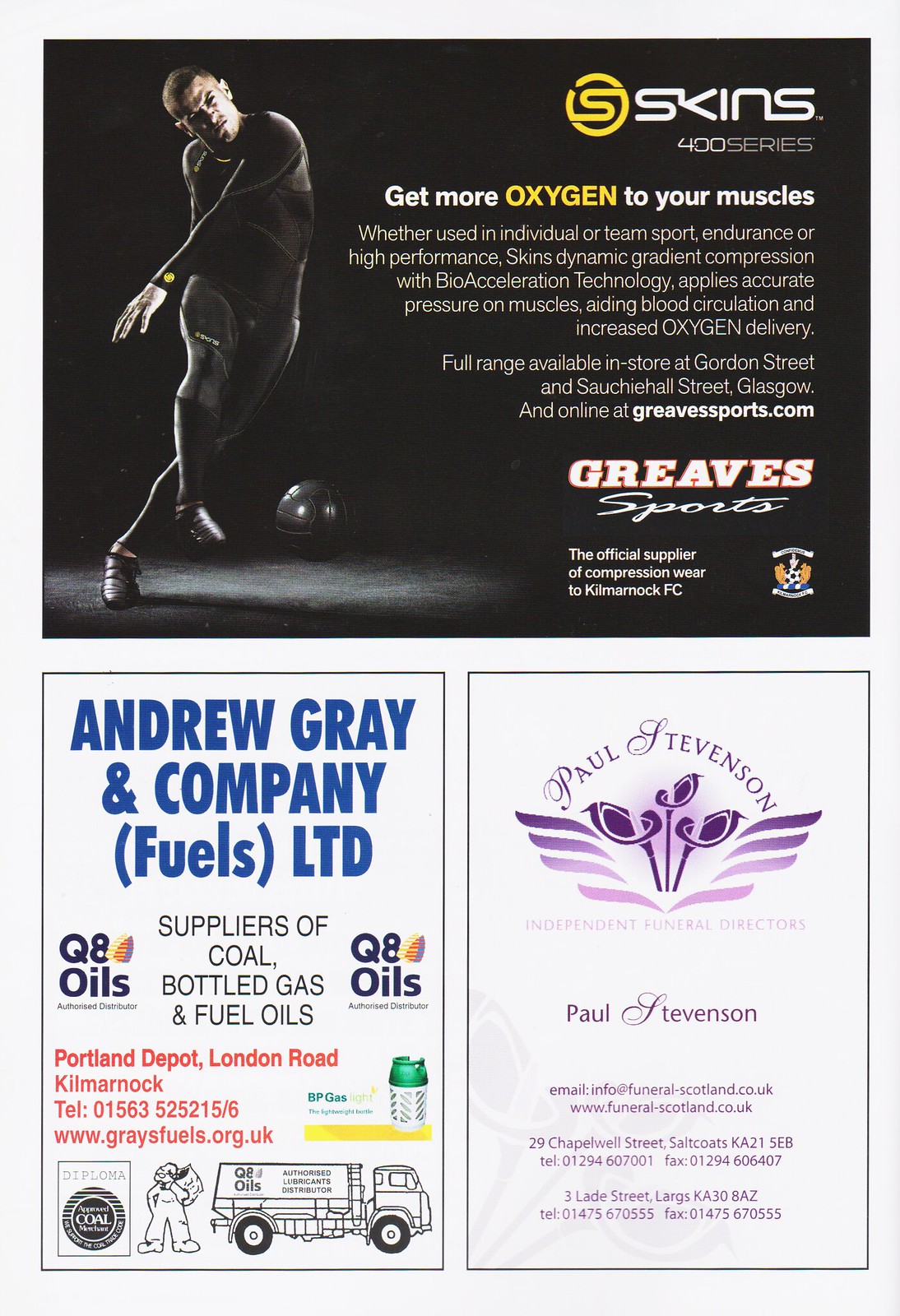The poster is a multi-colored print composed of four separate panels. The top third of the poster features a continuous, dramatic black background with a soccer player on the left, mid-kick, wearing a tight black skinsuit that enhances muscle oxygenation. The upper part prominently displays the Skins 400 Series logo alongside the slogan, "Get more oxygen to your muscles," emphasizing its use in both individual and team sports through Dynamic Gradient Compression technology.

Below this horizontal segment, the bottom portion is divided into two vertical panels. The left panel advertises Andrew Gray and Company, Fuels Limited, showcased with blue lettering detailing their services in coal, bottled gas, and fuel oils, accompanied by an illustration of a truck and a worker at the bottom.

The right panel features an image of purple lilies with a rainbow-like header reading Paul Stevenson in calligraphy, indicating his role as an Independent Funeral Director. The overall trim of the poster is white, framing these intricate advertisements.